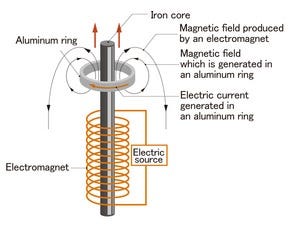This image is a detailed diagram of an electromagnetic component, specifically a 230-volt AC coil contactor. The background is plain with no borders, focusing solely on the illustrated components. At the center stands a silver rod, labeled as the iron core, which extends vertically. Around the lower to middle portion of this rod is a gold-colored coil, identified as the electromagnet and electric source. Toward the top of the rod is a silver ring, labeled as the aluminum ring.

Multiple labels and arrows annotate the various parts and their functions. The diagram features orange arrows pointing upwards from the iron core, explaining the production of a magnetic field by the electromagnet. Within the swirl representing the magnetic field, labels indicate the magnetic field and electric current generated in the aluminum ring. An additional swirl with arrows demonstrates the direction of the magnetic field within the aluminum ring, creating a comprehensive visual representation of the electromagnetic processes involved.